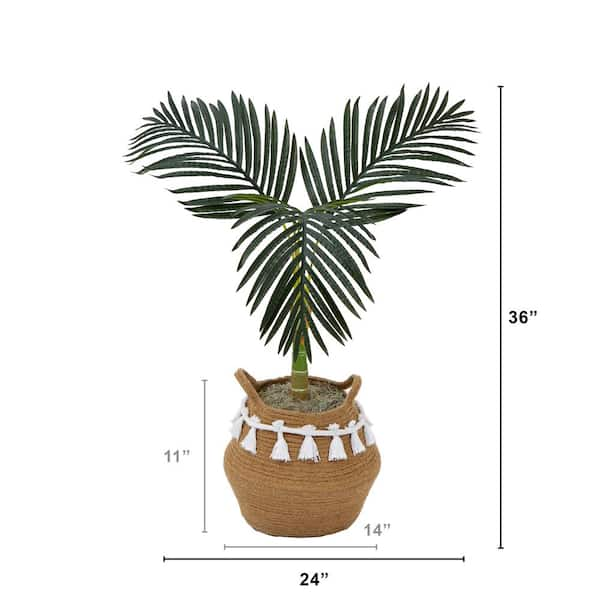This image features a palm-like plant with three long, thin fronds displaying evenly spaced green and white stripes. The plant stands inside a brownish, woven basket with white tassels dangling around its edges. Measurements are highlighted across different parts of the image, showing the overall height of the plant and pot together as 36 inches, the entire width of the plant and pot as 24 inches, the pot's height as 11 inches, and the pot's width as 14 inches. The background of the image is white, offering a clear and detailed view of the dimensions and the plant's structure.